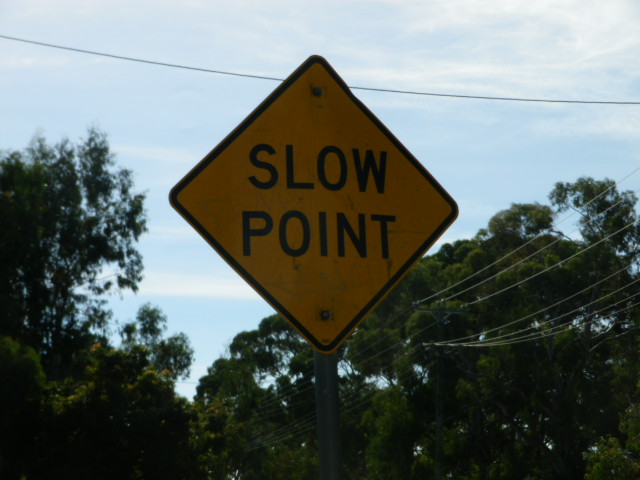This vibrant photograph captures a bright yellow, diamond-shaped street sign mounted on a sturdy metal pole, secured visibly by rivets. The sign stands against a picturesque backdrop, displaying the words "Slow Point" in bold black letters. Above and beyond, the sky is a brilliant azure, dotted with soft, fluffy white clouds. The scene is further enriched by lush green trees brimming with leaves, hinting at a serene shoreline or ocean in the distance. Adding to the rustic charm, telephone poles with wires stretch across the right side of the image, complemented by a prominent black wire cutting across the top portion of the frame.